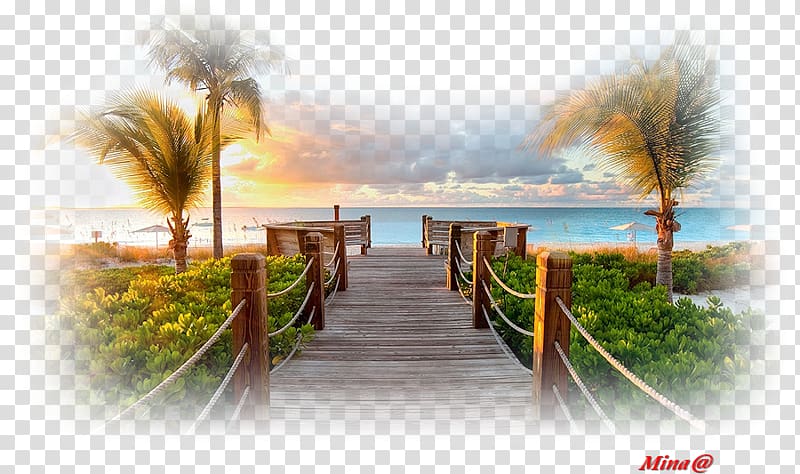In this detailed photograph of a tropical setting, we see a scenic raised boardwalk resembling a bridge, leading towards a beach and a clear blue ocean. The boardwalk, which features three levels of ropes strung between thick, heavy wooden posts, gently curves towards an open round area with potential seating, before descending to the sandy beach. Palm trees line both sides of the walkway amidst verdant green foliage. The background is marked with the setting sun near the horizon, casting a warm glow over the landscape. Large, square beach umbrellas are scattered along the water’s edge, with distant boats or people faintly visible in the ocean. Above, a mix of large clouds looms across the sky, suggesting an impending storm. The edges of the photograph are feathered, with a checkered pattern representing a clear alpha layer, and the name "Mina" followed by an at sign (@) is noted at the bottom right corner, possibly crediting the photographer.